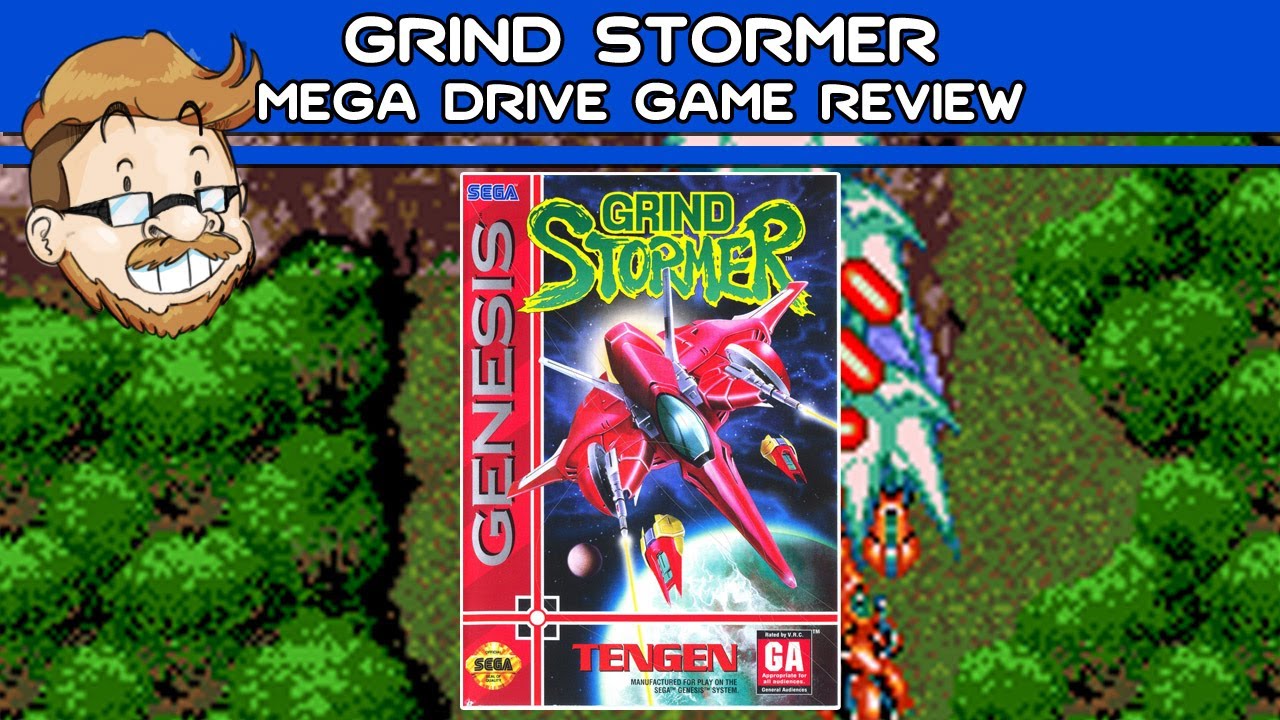The image resembles a YouTube thumbnail featuring an in-depth review of the Sega Genesis/Mega Drive game "GrindStormer." At the top, the thumbnail clearly displays a blue banner with the white text "GrindStormer Mega Drive Game Review." To the left is an illustrated, cartoon-like portrait of a man. The man has tan skin, black-framed glasses with a turquoise tint, a brown mustache, a brown beard, and light brown hair with a shaved style on the sides. He appears to be grinning.

The background of the image showcases an 8-bit style video game scene, depicting trees along the edges and green grass in the center, where a red spacecraft is prominently displayed, reminiscent of classic video game box art. This box art features the title "GrindStormer" in dark green letters with a yellow border at the top. A red banner on the left says "Genesis" in dark gray letters, and at the bottom, it reads "Sega" in blue, "Tangon" in a gold emblem, and "Genesis" once again in silver. The entire composition is laid out horizontally, providing a nostalgic and detailed visual summary of the game review.